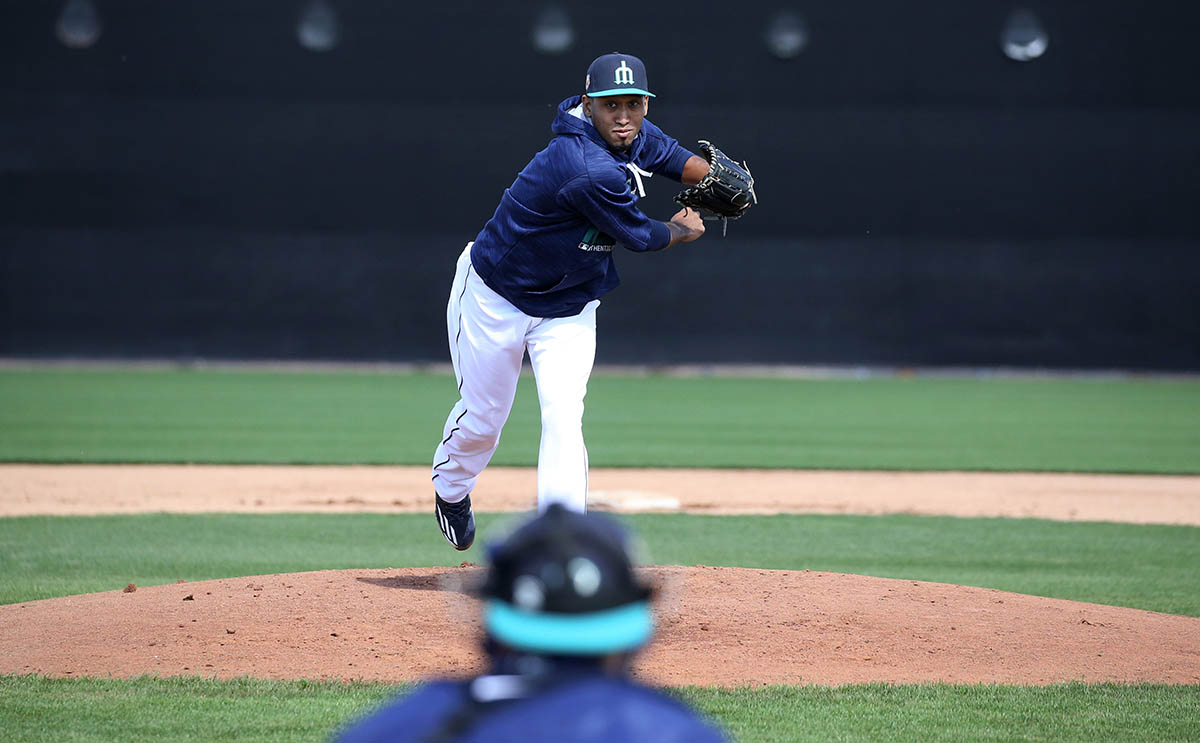In the image, we see a baseball game centered around a pitcher who has just completed a throwing motion. The pitcher is wearing a full blue uniform, including a blue hoodie and a cap with a distinctive logo resembling an upside-down set of three candles or an inverted pitchfork. His right arm is crossed over his body, suggesting he has just thrown the ball, while his left hand holds a black glove. He is also dressed in white pants with a stripe down the side and black shoes. The scene captures the pitcher standing on the mound with the baseball field in the background. There is a black background surrounding the field, indicating the outfield wall or an empty stadium. The blurred outline of the catcher is visible at the very bottom of the image, underscoring that this moment is focused on the pitching action, possibly during a warm-up or practice session. There is no text or visible team identifier beyond the logo on the pitcher's cap.